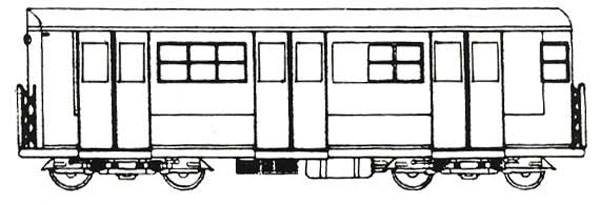The image is a black and white pencil drawing of a single train car, meticulously rendered with architectural precision. The train car is depicted with straight lines and circles, featuring double doors at the front, middle, and back sections. There are train track wheels at the front and back, two sets each. The middle section, beneath the double doors, has a fuel tank or similar structure. The front of the car displays two windows, while the middle section has two windows and a slider window. Additionally, there is a six-panel window located between the middle and back doors. The roof of the train car is rounded and contains a bar or guardrail at one of the entrances on the left side. Though the drawing appears basic and lacks intricate detail, the clear lines and framed grid windows effectively convey the concept of the train car. The image background is white, highlighting the black and white drawing style, reminiscent of a CAD design or a traced sketch.